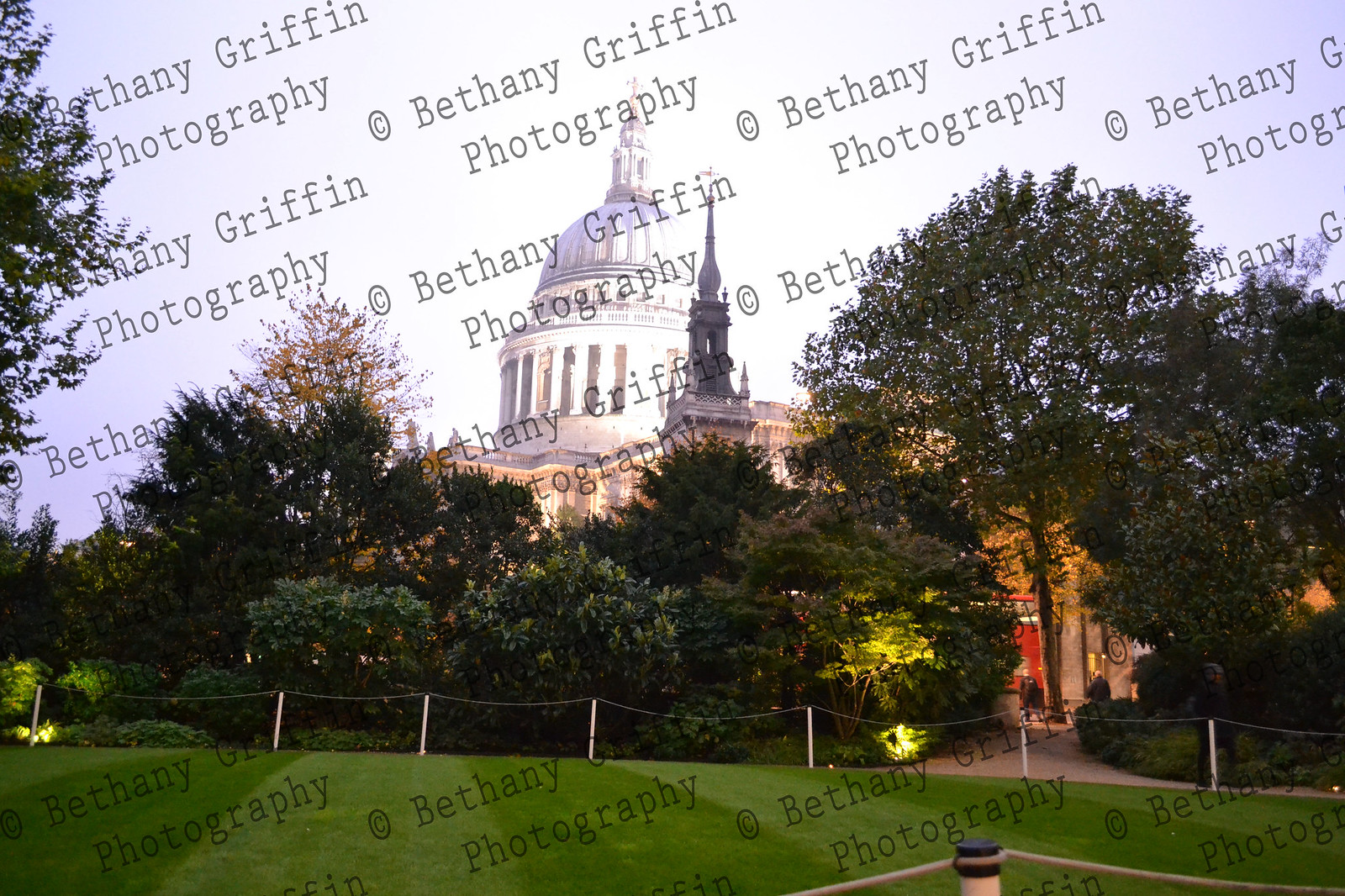This image captures an outdoor view of the Capitol building from the lawn. In the distance, the iconic white dome and spire of the Capitol are distinctly visible, glowing against a very white and clear sky, suggesting early evening. The middle ground is densely populated with various trees, hedges, and shrubs, partially obscuring the view of the building. The foreground features a neatly trimmed, striped green lawn, separated from the walkway by a rope fence supported by white posts. Scattered small lamps illuminate the path, adding to the scene's serene charm. A watermark text, "Copyright Bethany Griffin Photography," is repeatedly overlaid across the entire photograph, indicating the photographer's credit.